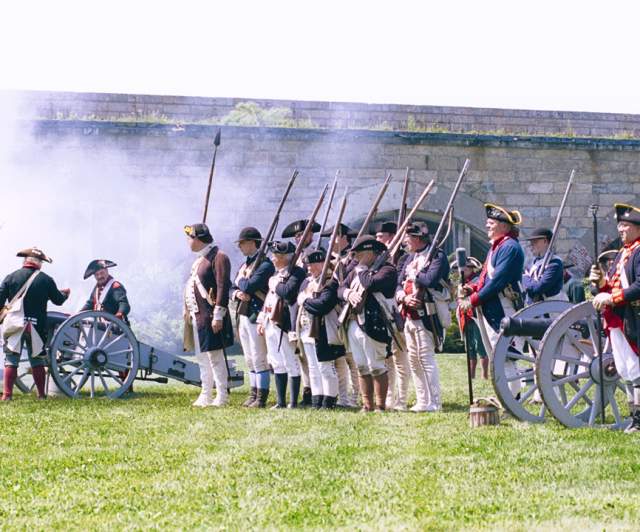This photograph captures an outdoor re-enactment of a Revolutionary War scene on a bright, sunny midday. The central focus is a group of soldiers dressed in distinctive Revolutionary War attire: white pants, shirts, and dark blue coats. They are arranged in formation, many holding muskets, while one prominent figure at the front brandishes a long spear. The backdrop features a large, natural stone fort with an arched walkway and a manicured grassy field. To the sides, additional soldiers stand by two cannons with large white wheels, from which smoke billows, likely from recent firing. The scene, marked by historical costumes and weaponry, evokes a vivid and detailed portrayal of a bygone military era.